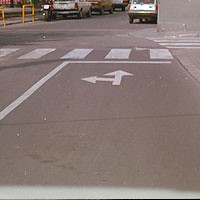The image captures a street view from the perspective of a driver looking through a windshield. The central focus is a lane with a white directional arrow painted on it, pointing both straight ahead and to the left. The lane approaches a prominent crosswalk marked by large yellow bars extending from the right to the left at the top of the image. Just before the crosswalk, there is a stop line and another solid white line to the left, dividing the lanes. Up ahead, a car is visible on the road, while on the left side, several cars are parallel-parked along the curb. Additionally, there's a second crosswalk on the far right side of the image, perpendicular to the main crosswalk. The overall scene is detailed with the street elements clearly marking out traffic directions and pedestrian areas.